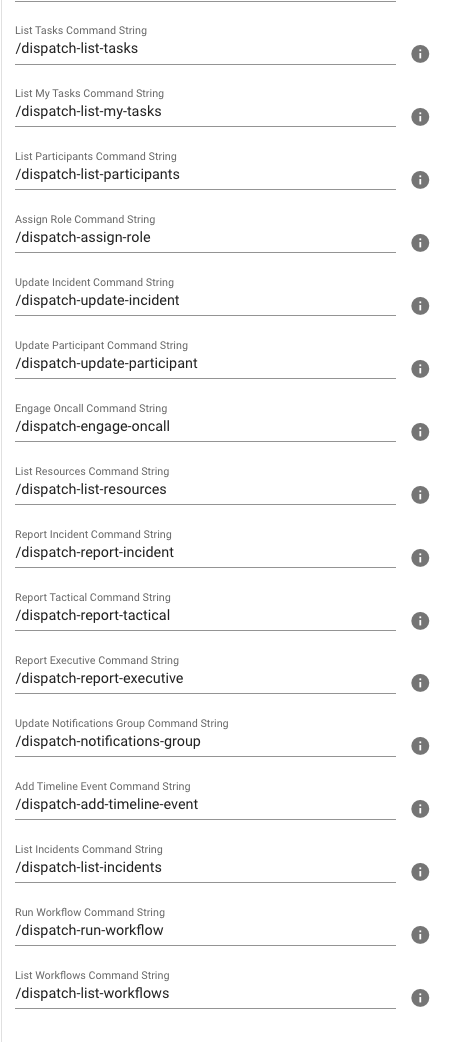This image is a screenshot of a webpage displaying command strings organized in a detailed and structured manner. The page is primarily divided into horizontal sections, resembling wide-ruled notebook paper, which neatly separates each line of commands. At the top of the page, written in small gray text, is the header "List Tasks Command String." Immediately below this header, the first command string is displayed in bold font as "\dispatch list tasks." Similarly, the second command string, labeled "List My Tasks Command String," is shown in bold as "\dispatch list my tasks."

For each command string, a corresponding category is listed in a column to the right, followed by specific types of commands underneath each category. Further to the right of each listing, there are gray circles containing a white eye icon, indicating visibility or additional details. The page uses divider lines between each entry, enhancing the organized, notebook-like appearance and making it easy to distinguish between different command strings. This meticulous layout ensures clarity and ease of understanding for users navigating through the command options.